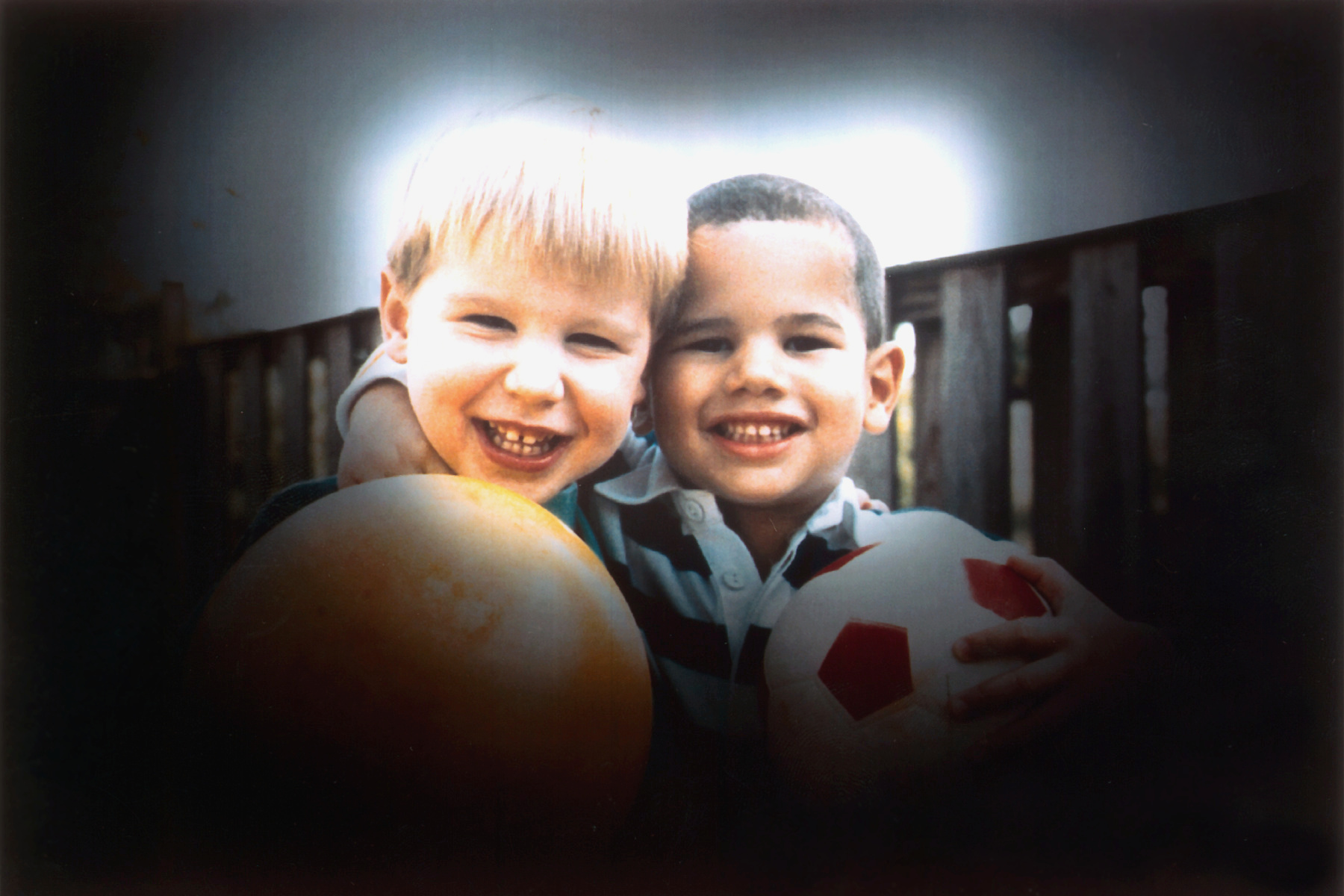In this photograph, two little boys around four years old are captured in a heartwarming moment of friendship, standing together in front of a brown wooden fence. The boy on the right has short, dark brown hair, brown eyes, and a darker complexion, possibly indicating he is Latino or Black. He is wearing a white and black shirt and affectionately has his arm around the neck of the boy on the left, who has medium blonde hair and lighter skin, and is dressed in a bright green shirt. Both boys are smiling joyfully at the camera, their teeth showing, and they seem to be enjoying each other’s company. The boy on the right is holding a white and red checkered soccer ball, while the boy on the left clutches a larger, orange ball with yellow and white accents. The photograph, likely taken in the 90s, features a vignette effect, making the edges very dark or even completely black, while the center is brightly illuminated, highlighting the boys' happy faces and colorful attire.